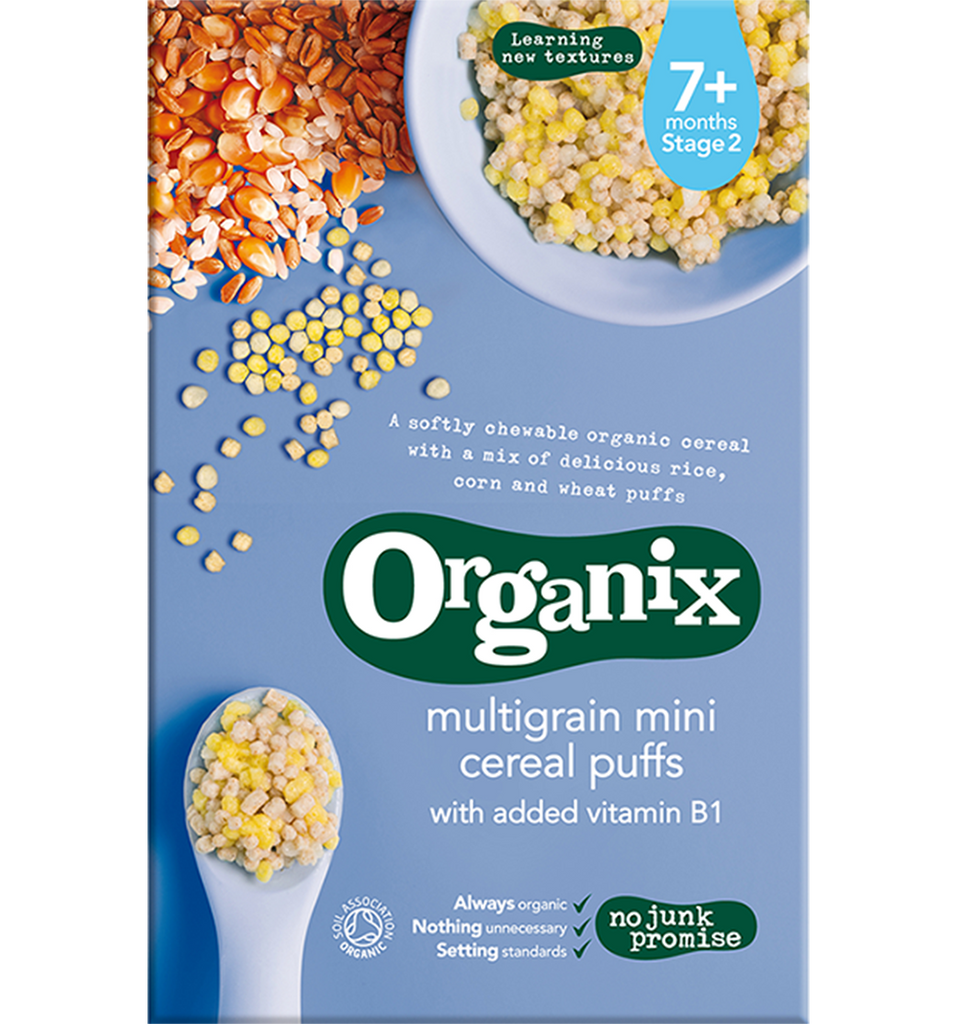The front of the cereal box features a light blue background with various detailed elements that highlight the product's qualities. At the top right, there's a white bowl filled with the cereal, consisting of small, colorful pellets that are a mixture of tan and yellow. The top left showcases corn and grains blending into the cereal. In the center of the box, "Organix" is prominently displayed in white text within a green, oval-shaped area. Above this, the text reads, "A softly chewable organic cereal with a mix of delicious rice, corn, and wheat puffs," while below it, "Multi-grain mini cereal puffs with added vitamin B1" is highlighted. There's also a checklist with green checkmarks stating "Always organic," "Nothing unnecessary," and "Setting standards," followed by a "No junk promise" mentioned within another green oval outline. Lastly, a spoon filled with the cereal is depicted on the left side, accentuating the cereal's texture and ingredients. The bottom left of the box contains a Soil Association organic logo alongside additional information, including a blue icon with a white number "7+" indicating the cereal is suitable for stage two of infant nutrition.